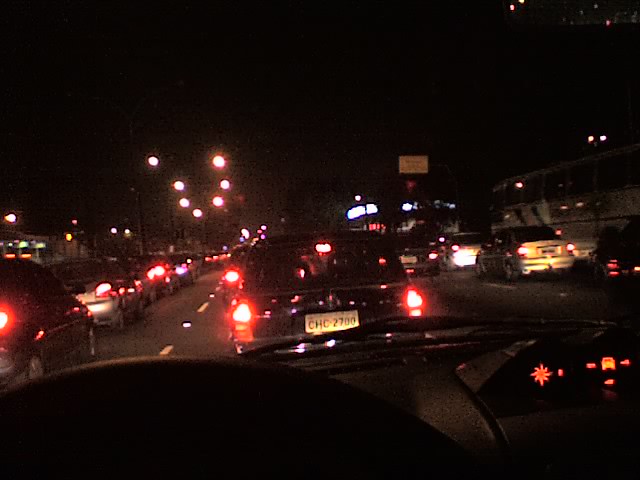A nighttime photograph taken from the driver's seat of a car captures the view through the windshield of a gridlocked four-lane highway. The scene is marked by bumper-to-bumper traffic, with rows of vehicles stretching into the distance. The driver is in the second lane from the left, surrounded by cars with glaring red brake lights, indicating a complete standstill. Ahead, a black sedan with the license plate CHC 2700 is visible. Streetlights illuminate the dark sky, and additional details include a white bus or train on the far right side of the road and some billboard street signs in the distance.